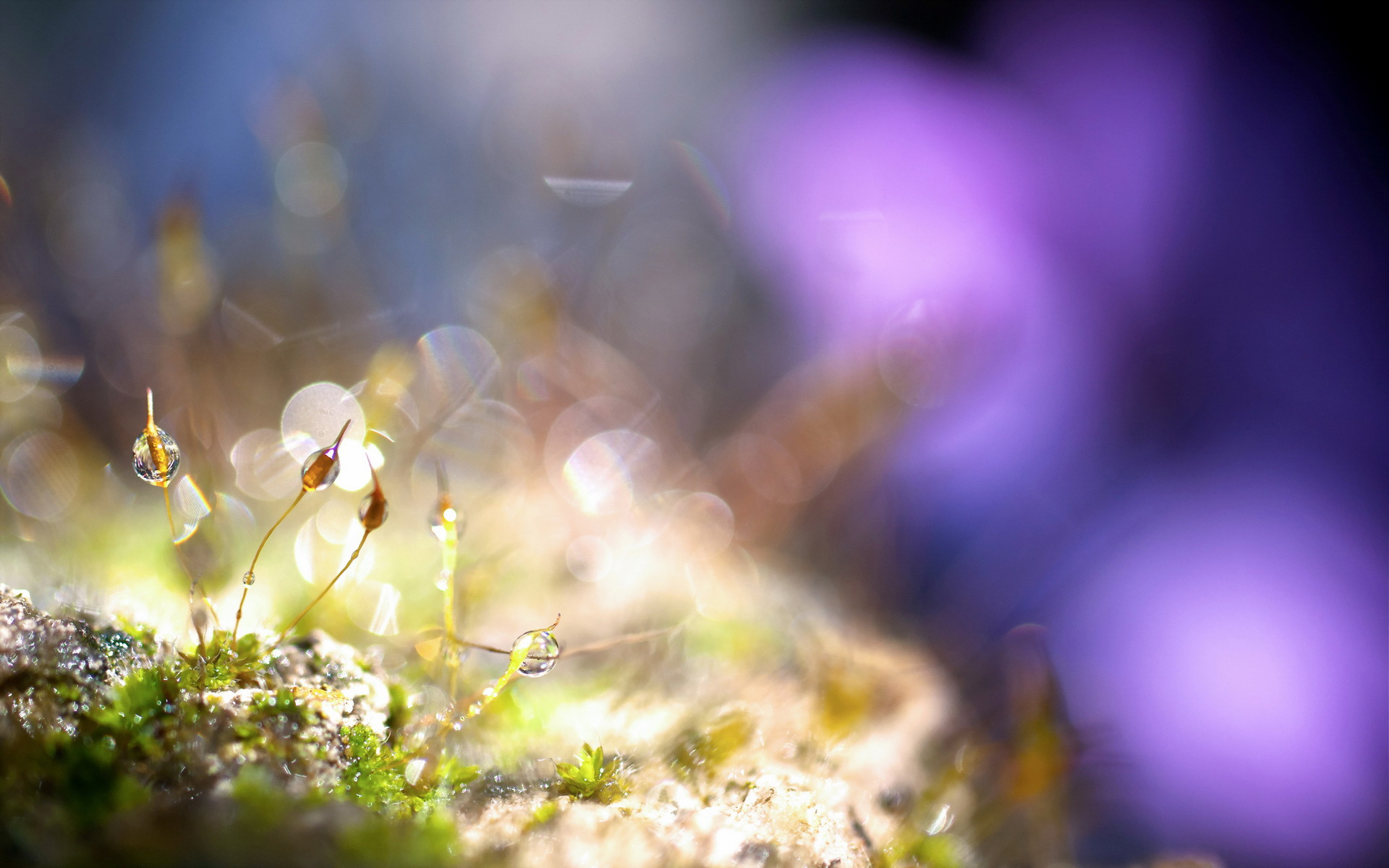The image showcases a close-up view of delicate plants adorned with dewdrops, glistening beautifully in the sunlight. These plants are growing on a textured, mossy surface that adds depth and contrast. A stunning interplay of light and shadow creates an ethereal, magical atmosphere. The background is softly blurred, featuring a harmonious blend of purples and blues that enhance the photo's overall quality. The focal point is a particular plant on the left side, where several dewdrops hang from its fine stems, all illuminated by natural light. Additionally, the scene includes lens flares and shimmering light reflections, with distinct light sources adding to the surreal feel of the image.